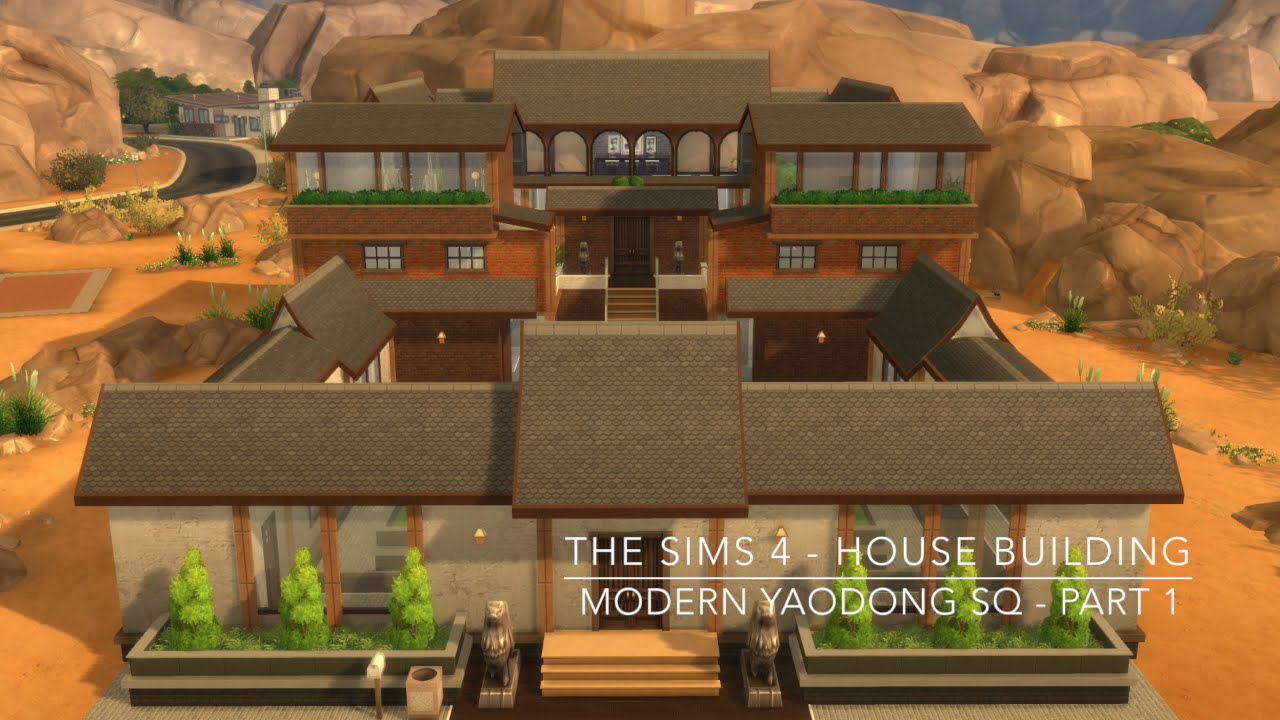The image depicts a detailed scene from the video game "The Sims 4," specifically titled "House Building: Modern Yaodong Square, Part 1." The focal point is a large, modern two-story house with a distinct architectural design. The house features a prominent entrance flanked by lion statues and three steps, leading to a triangular roof with white walls and a grayish facade. Surrounding the entrance is a small garden with three triangular-shaped plants. To the left and right of the entrance, there are gazebo-like coverings supported by pillars which delineate a square courtyard. Further back, another set of steps ascends to the main building. In the vicinity, one can also see a mailbox and a garbage can towards the left, along with a backdrop of brown mountains and a clear sky, enhancing the scenery. A road and another house are visible in the distance, complementing the game environment's realistic detail.